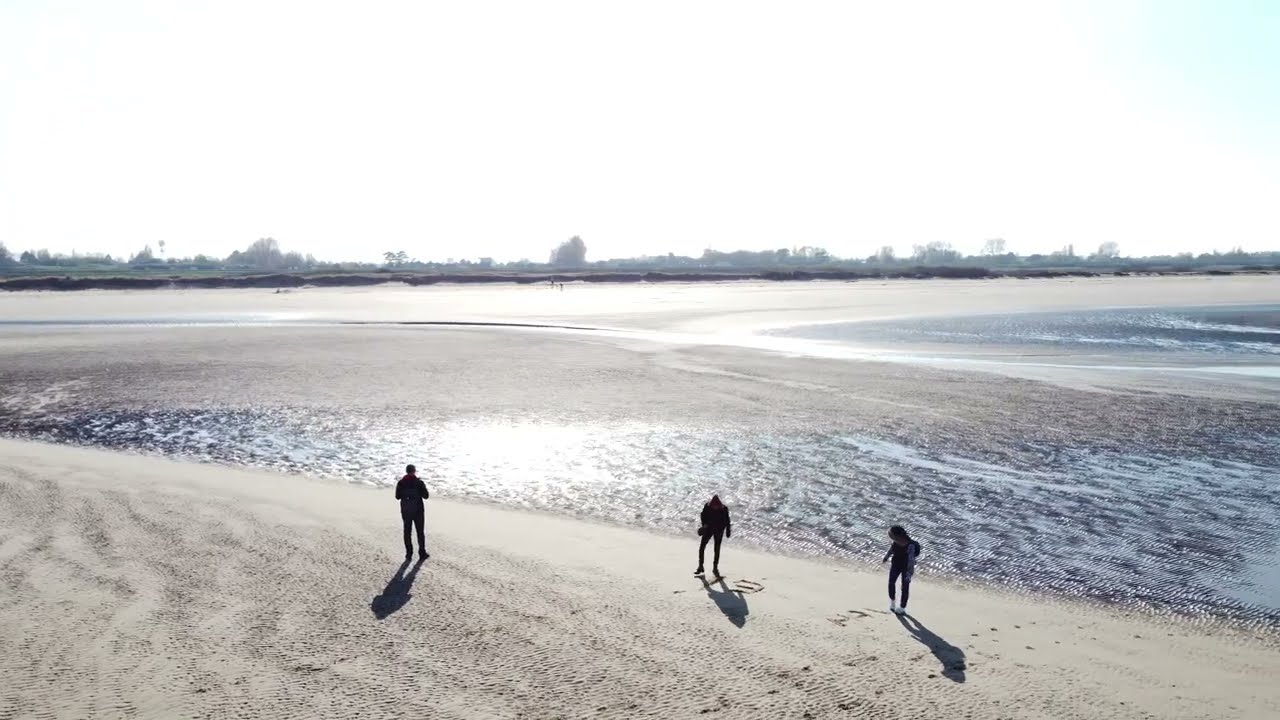In this landscape-style photo captured at low tide, three silhouetted individuals stand on a vast, reflective beach. The low tidal waters and expansive sandy shore stretch out under the bright, sunlit sky, which appears almost white due to the intense brightness. The sun illuminates from the horizon, casting long shadows of the individuals towards the camera and reflecting off the shallow waters. The figures are evenly spaced about 10 feet apart, with two on the right seemingly spelling out something in the sand with their feet, while the one on the left gazes out over the sparse, rippled water. In the distant background, faint outlines of trees, buildings, and dunes can be seen, adding depth to the serene, sun-drenched scene.